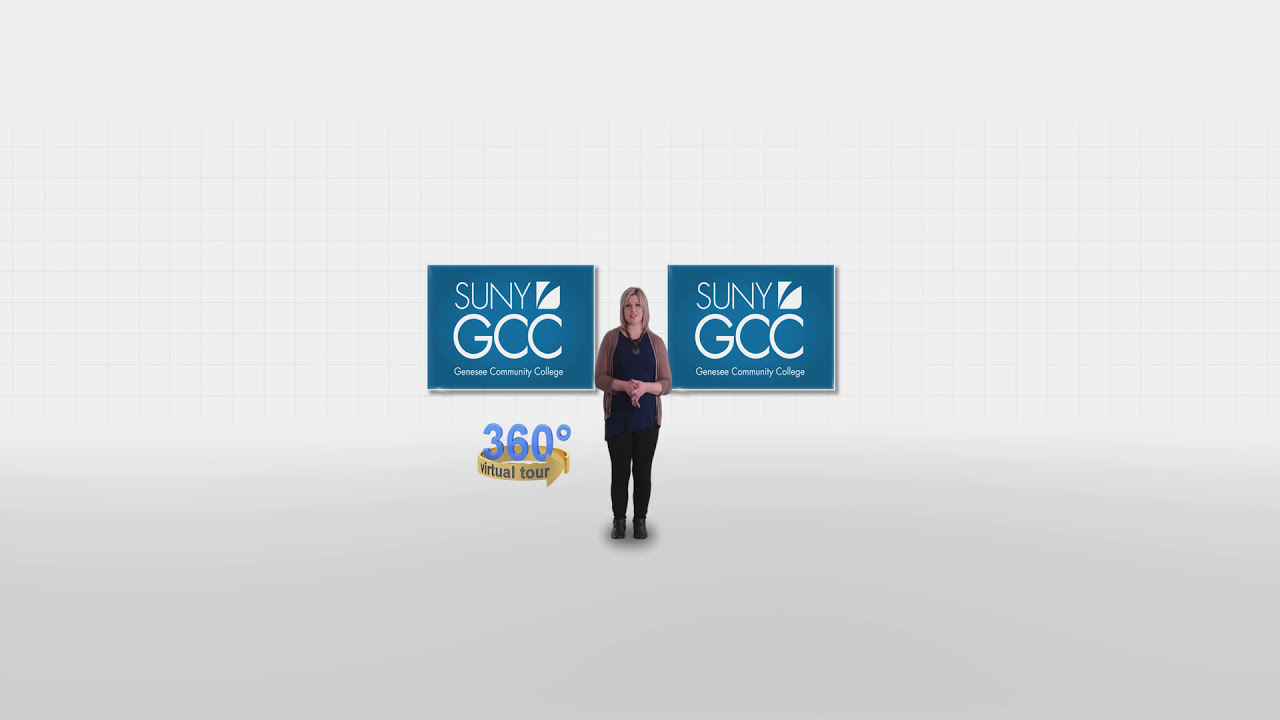The image appears to be an advertisement for Genesee Community College (SUNY GCC). It features a light gray background divided into two sections: the lower 40 percent is a slightly darker gray, while the upper 60 percent has a faint checkerboard pattern. Centered in the image is a woman with shoulder-length blonde hair, wearing a black blouse, black pants, and an open brown cardigan. On either side of her are identical teal logos for SUNY GCC, with the text "Genesee Community College" underneath. Notably, on the left side of the image, there is blue text reading "360 degrees" above a golden circular arrow with the words "Virtual Tour" inscribed within it. The woman appears to be facing and interacting with the camera, giving the impression this could be from a website's homepage.